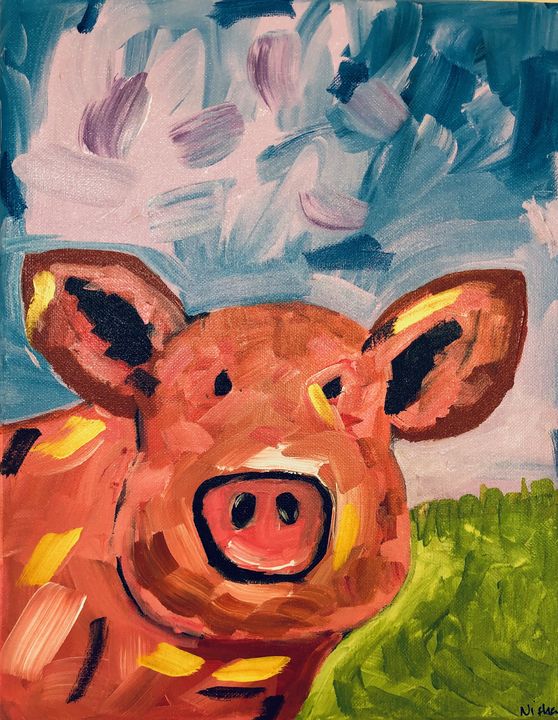This vivid painting creatively depicts a pig composed of colorful splotches and thick brush strokes that resemble finger painting. The pig, characterized by its pink, orange, yellow, black, and peach hues, stands out against a vibrant background. The animal's snout and ears are distinctly pig-like, and it gazes straight ahead with a somewhat questioning expression. The setting includes a green field, portrayed with varied shades from lime to hunter green, and a sky filled with white, blue, and hints of purple smudges. Despite its stylized, non-realistic approach, with every feature splotched and smudged into life, the painting unmistakably captures the essence of a pig. A barely legible signature with the letters "N" and "I" followed by a squiggle appears at the bottom, adding a personal touch from the artist.